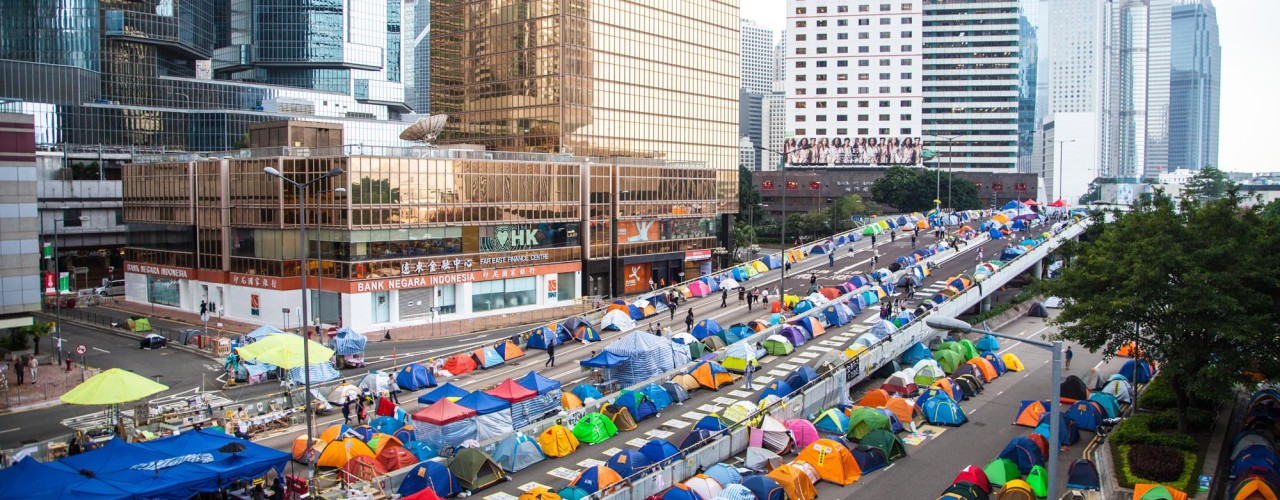The image depicts a bustling street scene in what appears to be an urban area in Indonesia, suggested by the presence of signage such as "Bank Negara Indonesia" and some Chinese characters. The road is slightly slanted upwards, covered with a variety of brightly colored tents—orange, dark blue, blue, pink, white, yellow, black, red, teal, and more—that seem to serve as shelter for homeless individuals or people displaced by a disaster. These tents are haphazardly placed on the street and some spill over onto the sidewalk. The background features numerous tall buildings, indicating a dense urban environment. On the bottom right corner of the image, a large tree is visible next to a streetlight, adding a touch of greenery to the otherwise crowded and chaotic street scene.